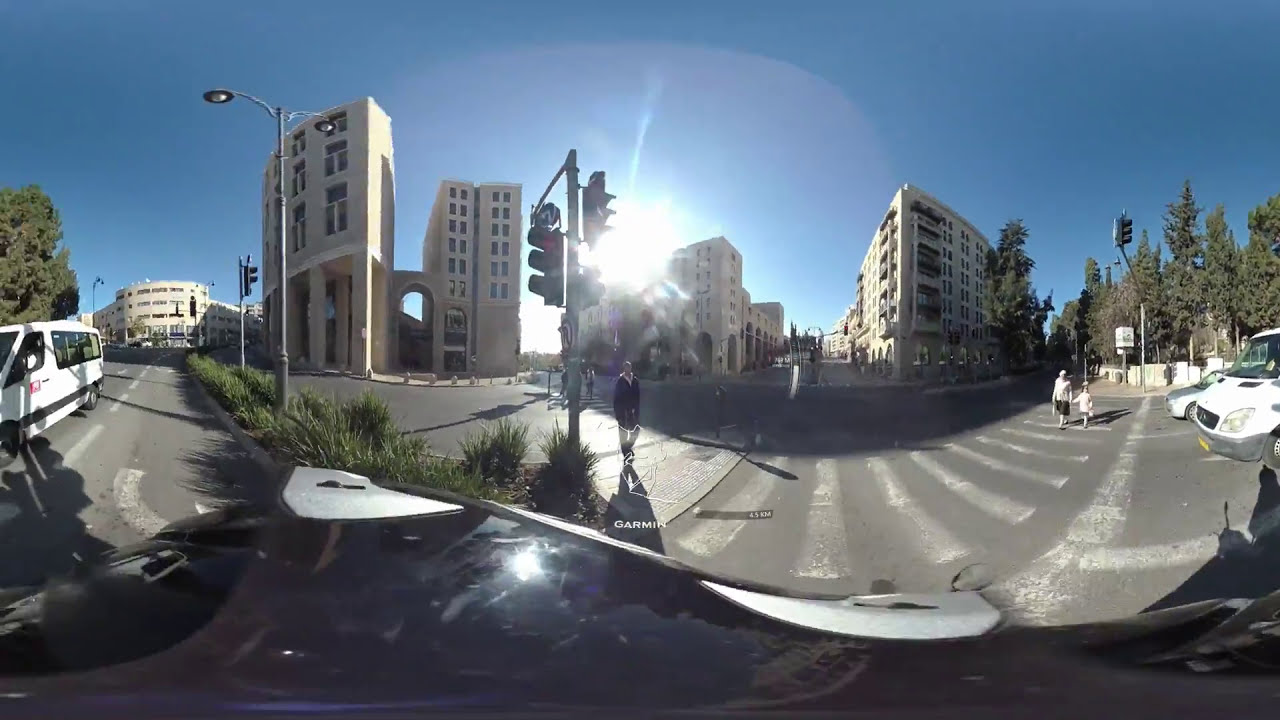In the foreground of this clear, sunny day, a vibrant urban scene unfolds with people crossing a busy intersection in a modern European city. The cityscape is dominated by tall, white buildings, mostly commercial with a hint of residential apartments, featuring architectural arches connecting them. The scene is set against a backdrop of pine trees and a piercing blue sky. On the left side of the road, a white van approaches the camera, passing by a grassy area dotted with a street lamp and a stoplight. Meanwhile, on the right side, parked white vehicles line a roadway near a parking area where a woman walks with a young girl. At the center, possibly downtown, traffic lights oversee the intersection, while the roads converge in the distance. The city view is slightly warped due to the 360-degree nature of the image, allowing multiple perspectives of the same car. The golden sunlight, suggesting early morning, floods the scene, enhancing the vividness of the bustling urban atmosphere.